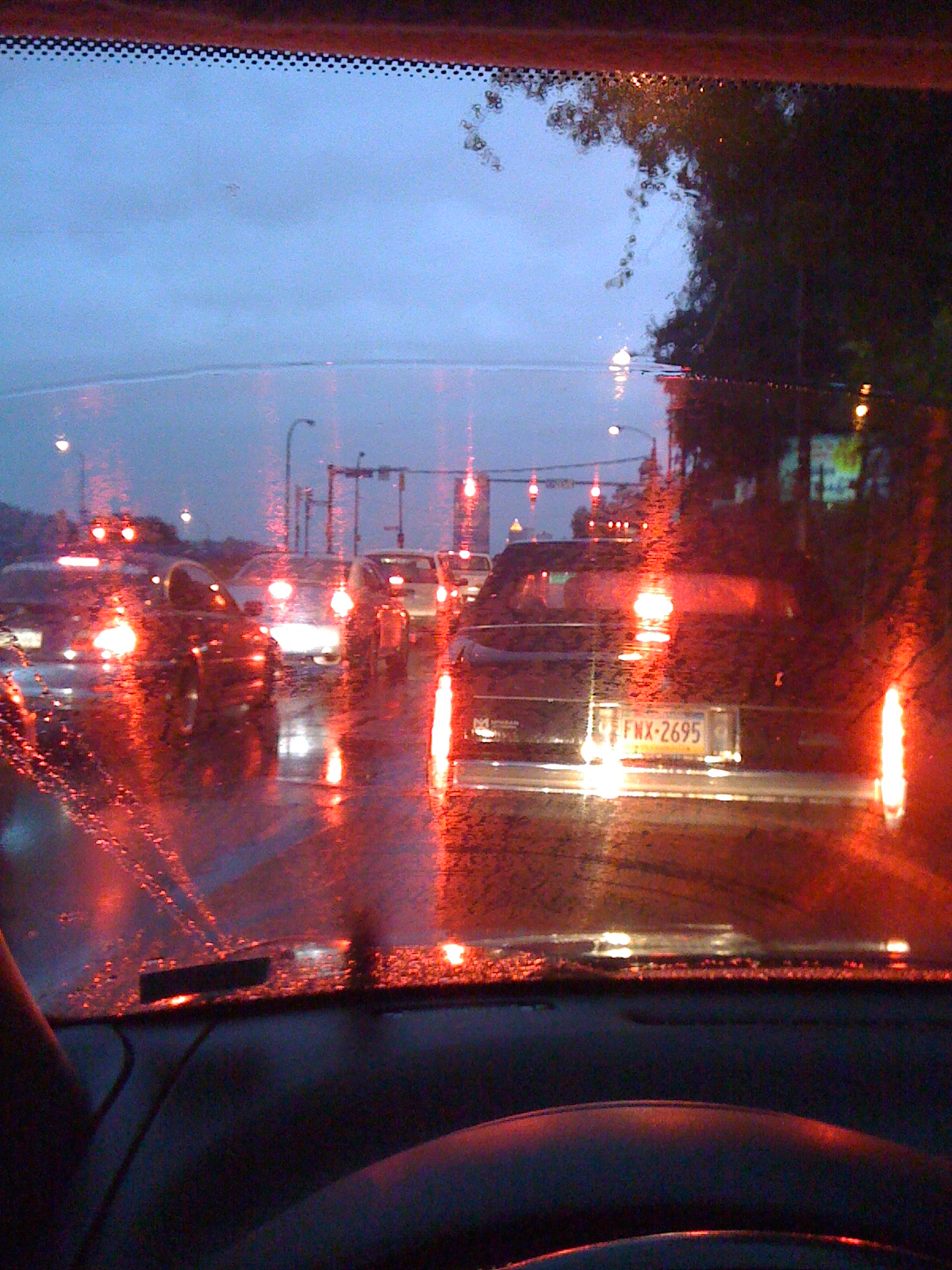This image captures a driver's perspective, viewed through the windshield of a car at nighttime or possibly dusk, with a hint of rain evident from the water streaks and glare on the glass. The dashboard is visible at the very bottom, showcasing a gray surface. Ahead, the scene is dominated by a large, black luxury vehicle with its brake lights glowing red. To the left, a parallel lane of cars also displays their illuminated brake lights, suggesting the driver is in the midst of traffic.

The night sky is a gradient from dark blue to a lighter blue at the center, while the upper part of the image presents the interior roof of the car. On the right side, the outline of a tree's overhang partially obscures a distant billboard sign with a white base and a yellow circle. Several streetlights and telephone poles can be seen further ahead, with the distant traffic lights all appearing red, emphasizing the traffic halt. The combination of brake light reflections on the wet windshield and the streetlights creates a vivid, atmospheric scene of an evening or nighttime drive in traffic.